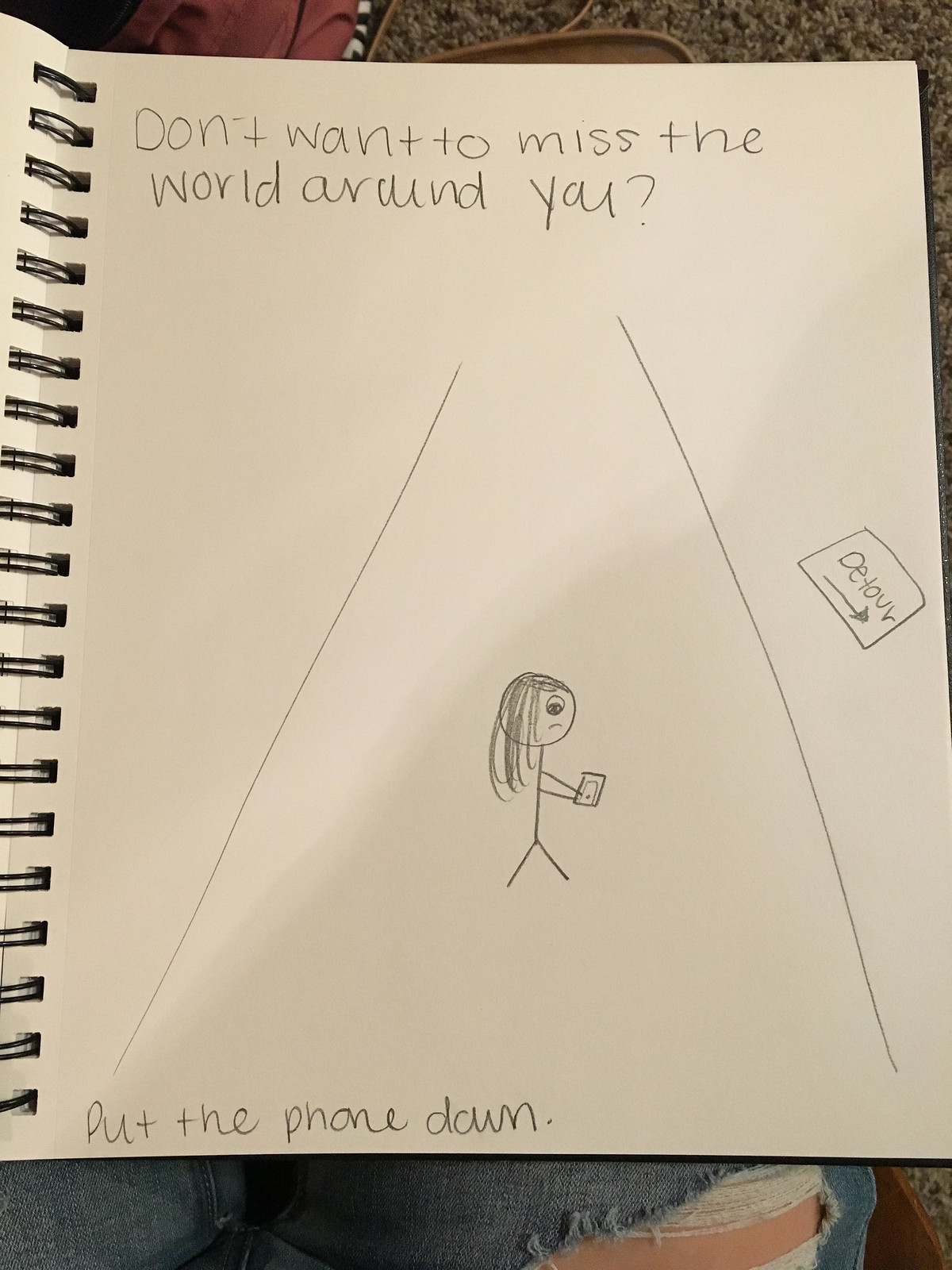This photograph captures a detailed pencil drawing on a plain, unlined sheet of paper within a spiral-bound sketchbook. The sketchbook rests on someone's legs, clad in blue jeans with a visible tear on the thigh. At the top of the page, an ink caption reads, "Don't want to miss the world around you?" The center of the drawing features a stick figure girl with long hair holding a phone in her hands, illustrated walking between two parallel lines that represent a road, narrowing towards the top like a funnel. To the right side of the road, there is a sign marked "detour" with an arrow pointing downward. At the bottom of the drawing, another handwritten note in pencil advises, "Put the phone down." The artwork captures a poignant reminder to be present in the world around us, conveyed through its simple yet impactful imagery and text.